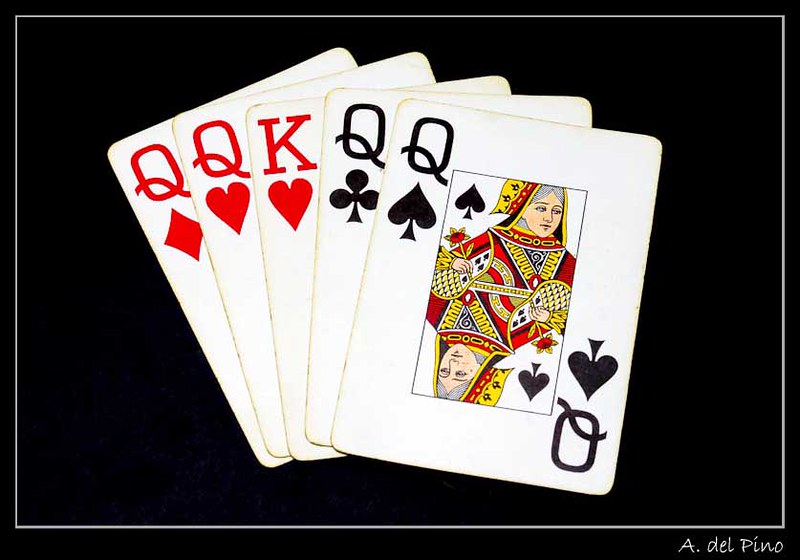This image features five slightly jumbled playing cards against a completely black background, accented by a faint, grayish-white border. In the bottom right corner, the artist's name, "a.delpino," is inscribed. The cards exhibit a well-used appearance with a subtle yellow tint along their edges, contrasting against their primarily white surface. Among the cards, three bear red suits while two are black. The top card is the Queen of Spades, prominently displayed. The other cards include the Queen of Hearts, the King of Hearts, and two additional queens, each adorned with the traditional illustrations found in standard playing decks.